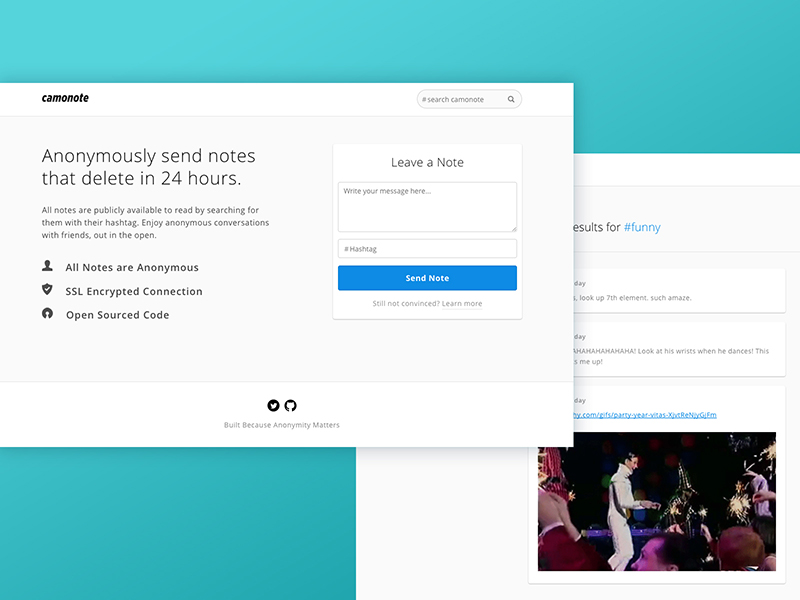As the sun sets and the battle comes to a grueling end, the scene captures the chaos and urgency of the moment. Soldiers are seen rushing towards a dropship, a critically injured comrade in their midst. One soldier, presumably Murphy, is being urgently instructed to roll the injured man onto his side, a precautionary measure taught by another soldier named Doug. The injured man's face is ashen, but he manages to utter reassurances to Murphy, who appears physically and emotionally exhausted. "You're okay, you're okay," he murmurs, his voice both soothing and desperate as he tries to stabilize him. 

Murphy's attention is fixated on the injured soldier, his hands trembling as he reassures, "All right, I got you, okay, okay, breathe. All right, listen, you and me are good. It's better." Despite the chaos around them, an intimate bond is clear between the two as Murphy gently places a hook around his neck, only to be met with resistance. "Why are you knocking me? Why not?" he questions, his voice tinged with confusion and desperation. Another soldier steps in, urging them to lay the injured man down properly.

In a heart-wrenching moment, the injured soldier looks up at Murphy, vulnerability in his eyes. "Hey, my brother," he whispers, his voice cracking with fear, "I'm scared." Murphy chokes back his own tears as he promises, "I won't let anything happen to you. I promise." The scene is filled with poignant tension, their brotherhood shining through in these dire circumstances. A quiet moment of levity is shared as the injured soldier, in a voice filled with pain but also a hint of humor, says, "I've never said shit to Tasia before." Murphy responds with a tired but genuine laugh, "You've told me that like a thousand times." 

The dropship looms closer, ready to take them away from the battlefield, but their connection and the gravity of the situation linger in the air, making it an emotional and evocative moment.